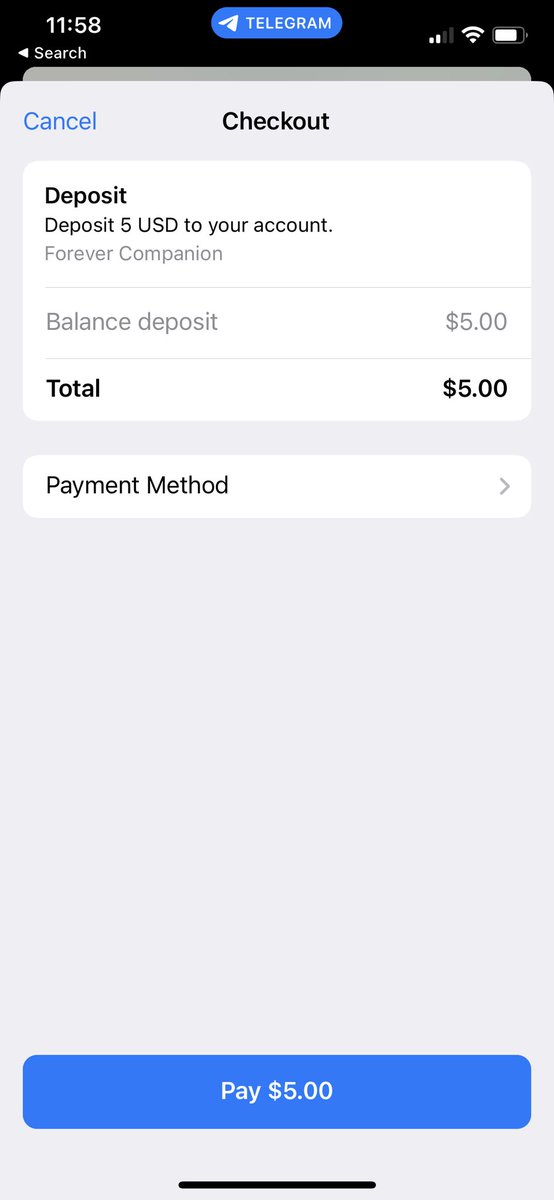A screenshot of a cell phone screen captured at 11:58 displays various interface elements and statuses. The phone has almost a full battery, its volume is maximized, but it shows a weak cellular signal. In the top center, the Telegram app is active, indicated by a blue highlight. The focal point of the screen is a transaction interface where the user is in the process of depositing money. The interface features a light blue-grey background with black text. A message reads "checkout," confirming a deposit of $5 to the user's account. The current balance and total deposit both display $5. At the bottom of the screen, there is an actionable button labeled "Pay $5," allowing the user to complete the money transfer.